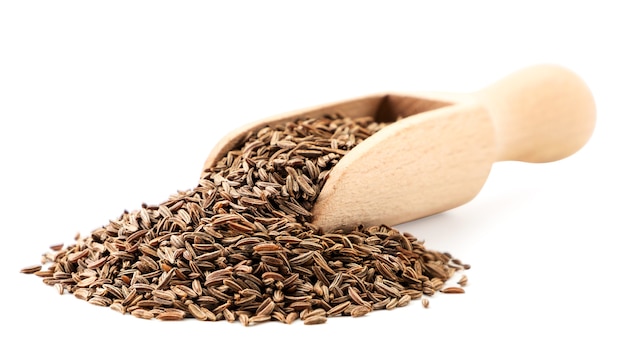The image depicts a light wooden scoop with a handle, placed on a white surface. The scoop is filled to overflowing with seeds that highly resemble sunflower seeds. These seeds display a variety of striped patterns in black, greenish, and tan hues. Many of them have spilled from the scoop, forming a neatly arranged circular pile in front of it. The scoop itself has a rectangular shape with rounded sides, and the handle, positioned at the top right of the image, features a rounded grip. The seeds are elongated and vary in size, highlighting the natural texture and color variations. The overall scene is clearly posed, emphasizing the natural beauty of the scoop and seeds against the stark white background.